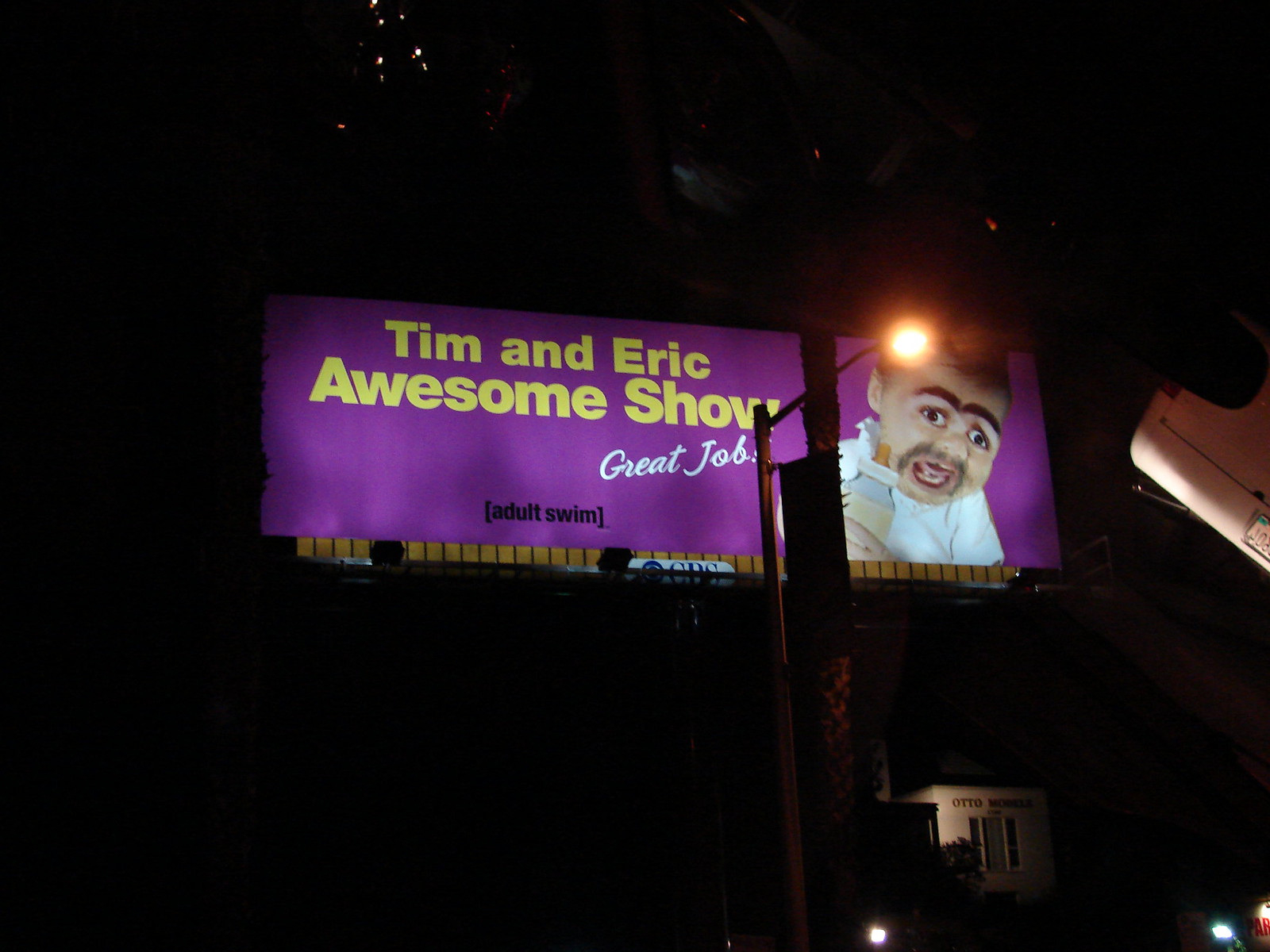The image captures a nighttime scene taken from inside a car, evidenced by the rear-view mirror and a white visor visible at the sides of the frame. The focal point is a brightly illuminated billboard featuring a promo for "Tim and Eric Awesome Show." The billboard stands against a backdrop of darkness, partially obscuring any surrounding details, though a street light and some partially illuminated building can be seen below.

The billboard itself has a striking purple background with the show's title "Tim and Eric" written prominently in yellow. Below that, in a cursive font and tilted slightly, it reads "does a great job." At the bottom-center of the billboard, the "Adult Swim" logo is clearly visible. The main visual element on the billboard is an amusing image of a man with a buzz cut, thick bushy unibrow, and a goatee, dressed in a white shirt. Interestingly, this man is holding a baby bottle instead of a microphone, adding to the quirky humor of the show. Additionally, there is a baby on the right side of the billboard, holding a bottle, further enhancing the playful and unusual aesthetic of the advertisement.